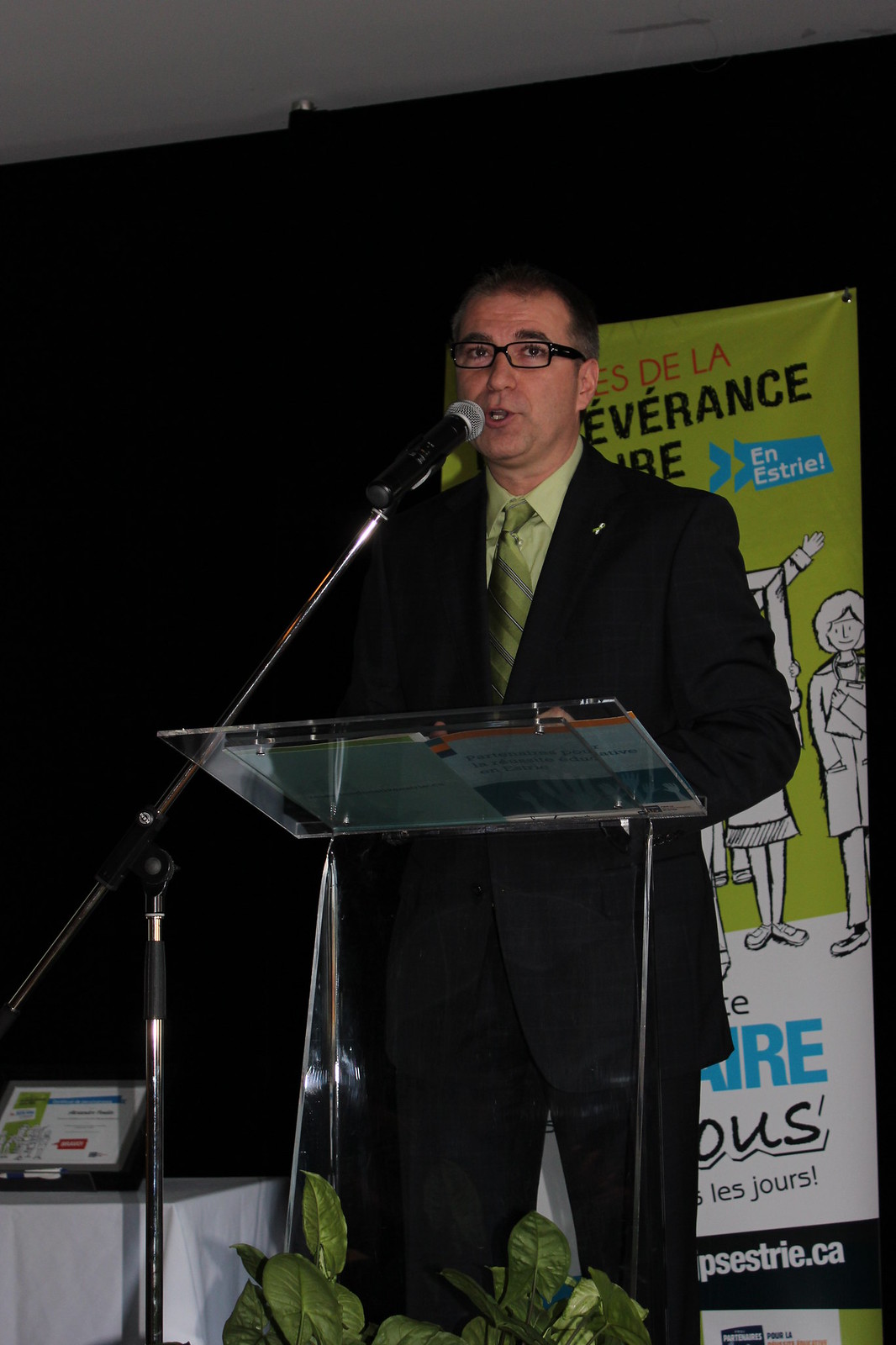In this photograph, a man in his 40s or 50s, possibly Latino, is captured mid-speech, addressing an unseen audience. Dressed in a black suit with an olive green shirt and tie, he stands behind a sleek, transparent glass podium that holds his guidebook. His short, buzzed hair and black-rimmed glasses frame his intent expression as he speaks into a black microphone mounted on a stand. The man is set against a dark backdrop, partially obscuring a lime green vertical banner adorned with illustrations of young people and text that appears to be in Spanish. Below the podium, a few green leaves from a plant are visible, adding a touch of greenery to the otherwise minimalistic scene.